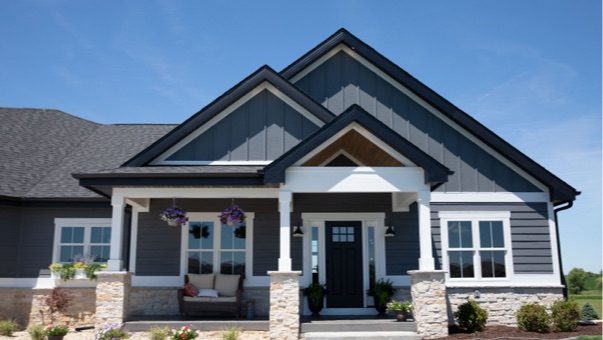This photograph showcases a single-story, modern American Craftsman-style house with a triple-roof design featuring overlapping triangular roofs. The house, bathed in daylight under a clear, blue sky, is painted in a striking blue-gray tone with dark gray accents and features both stonework and wood elements. The front porch, supported by two square-shaped pillars with stone bases and vertical wood beams, creates a welcoming overhang. The central navy door, adorned with six square windows, is flanked by side windows and planters. Surrounding the entrance is a landscaped garden with three boxwood bushes to the right and an assortment of flowers and long grasses to the left, all set against a stone mulch background. To the right of the porch sits a wicker loveseat, adding a cozy touch. Above the porch, hanging flower pots add a splash of color. The house has shake-style, brown roofing and showcases stonework at the lower part of the structure, about three feet high. The visible vegetation includes a green field with trees behind the house, and the bottom right corner of the image hints at the surrounding grass and greenery. Three front-facing windows with white borders likely provide light to the living room and perhaps a family room.